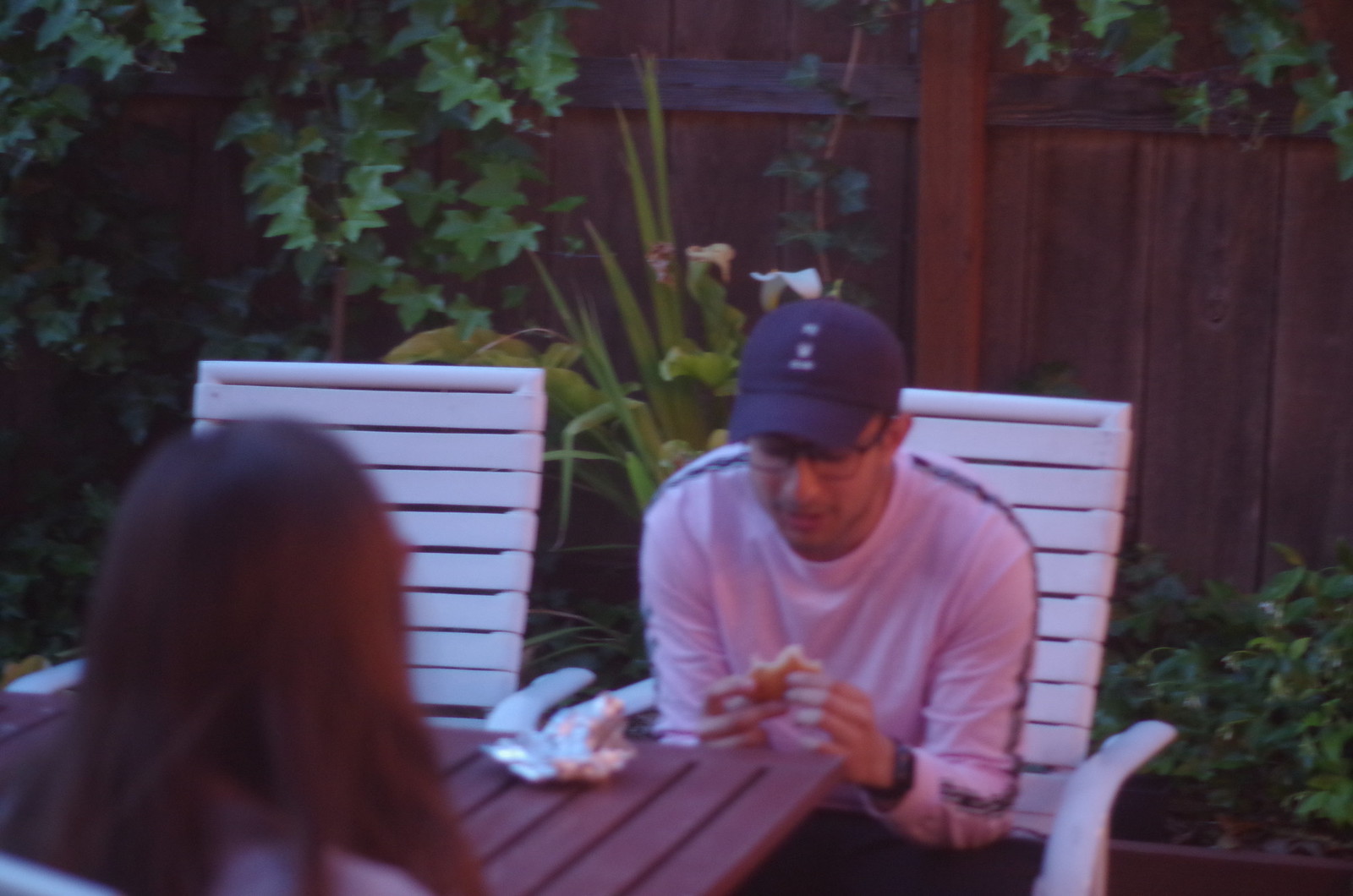In this photograph, two people are seated at a dark brown table in what appears to be a backyard or a fenced-in area. The composition captures the scene from behind a woman positioned in the bottom left corner, who has long brown hair cascading down her back. She faces a man directly across from her, identifiable by his white long-sleeve shirt, dark blue baseball cap, and glasses. He is in the midst of eating a sandwich with multiple bites taken out, which he holds with both hands. A tinfoil wrapper lies unfolded on the table, suggesting a casual, outdoor meal. The man sits comfortably in a white plastic chair, with an additional chair of the same type positioned to the left. The background consists of a brown wooden fence enveloped by lush greenery, including various trees, vines, and other plants, creating a serene natural setting for their gathering.